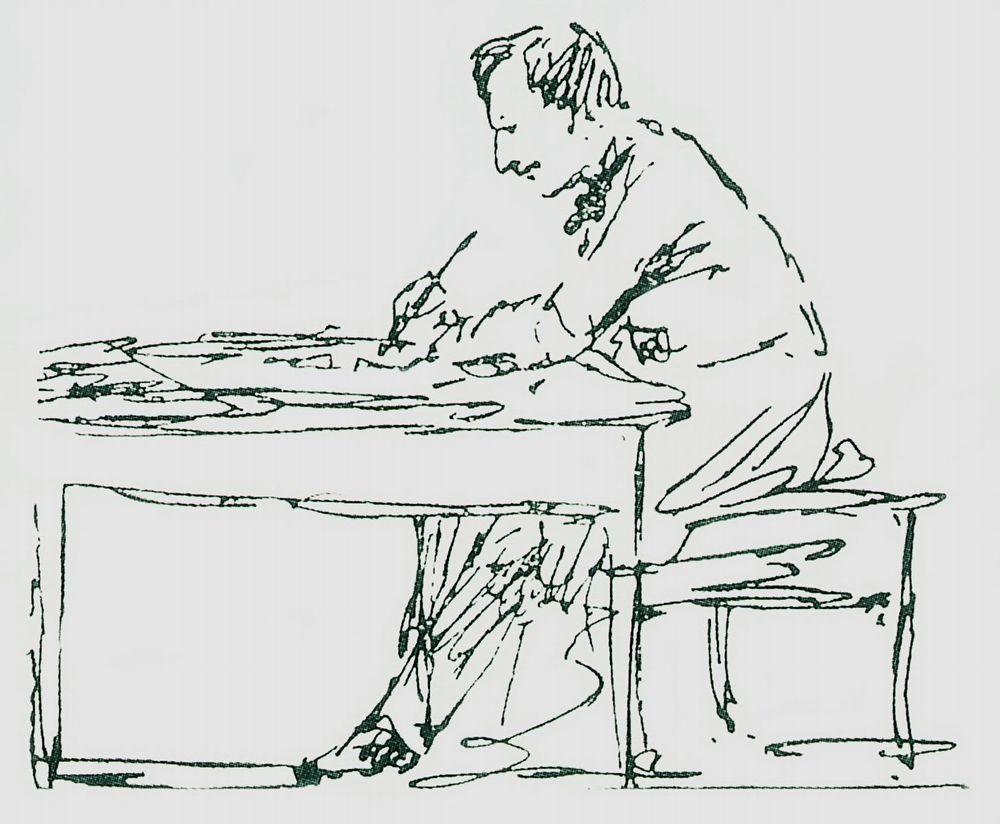The image is a monochromatic black and white pencil sketch, featuring the side view of a man centrally placed, meticulously detailed yet impressionistic in style. The man, impeccably dressed in a suit with what appears to be an ascot or bow tie, sits at a wooden desk. His right hand holds a quill or pen poised above a piece of paper, while his left arm rests on the desk. The desk, taking up the bottom left corner of the image and stretching towards the center, is accompanied by a neatly arranged stack of papers. The man himself is seated on a small wooden bench located in the bottom right-hand corner. The loose, expressive lines of the sketch suggest an indoor setting, likely the man's study. The overall composition is highly detailed, highlighting both the serene moment of creation and the minimalist, impressionistic artistic style.